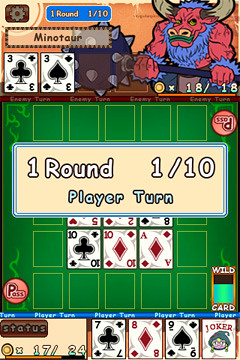The image is a colorful, detailed screenshot from a card game likely played on a mobile phone. Dominated by a vertically-oriented screen, the game board features a green baize grid table with cards arranged in a square pattern in the center. Visible cards on the grid include a five of hearts, a two of diamonds, an eight of spades, a ten of clubs, a ten of diamonds, and an ace of diamonds. 

At the bottom of the screen, the player's hand is displayed, containing a seven of clubs, an eight of diamonds, a nine of spades, and a joker card. The user interface indicates a counter for gold coins, showing 17 out of 24, and a turn indicator that reads "Round 1, 1 of 10, Play or Turn," with this information repeated both at the top and in a beige rectangle in the center of the screen.

The top section of the image features the opponent, a Minotaur avatar, characterized by pink skin, blue fur, and green lips, wielding a dark, spiky mace. The Minotaur, who has a three of clubs and a three of spades in his hand, is partially dressed in blue vest-like fur and blue bracelets. His coin counter shows 18 out of a total of 18 coins. The overall image appears to capture the essence of a strategic and visually engaging card game experience.